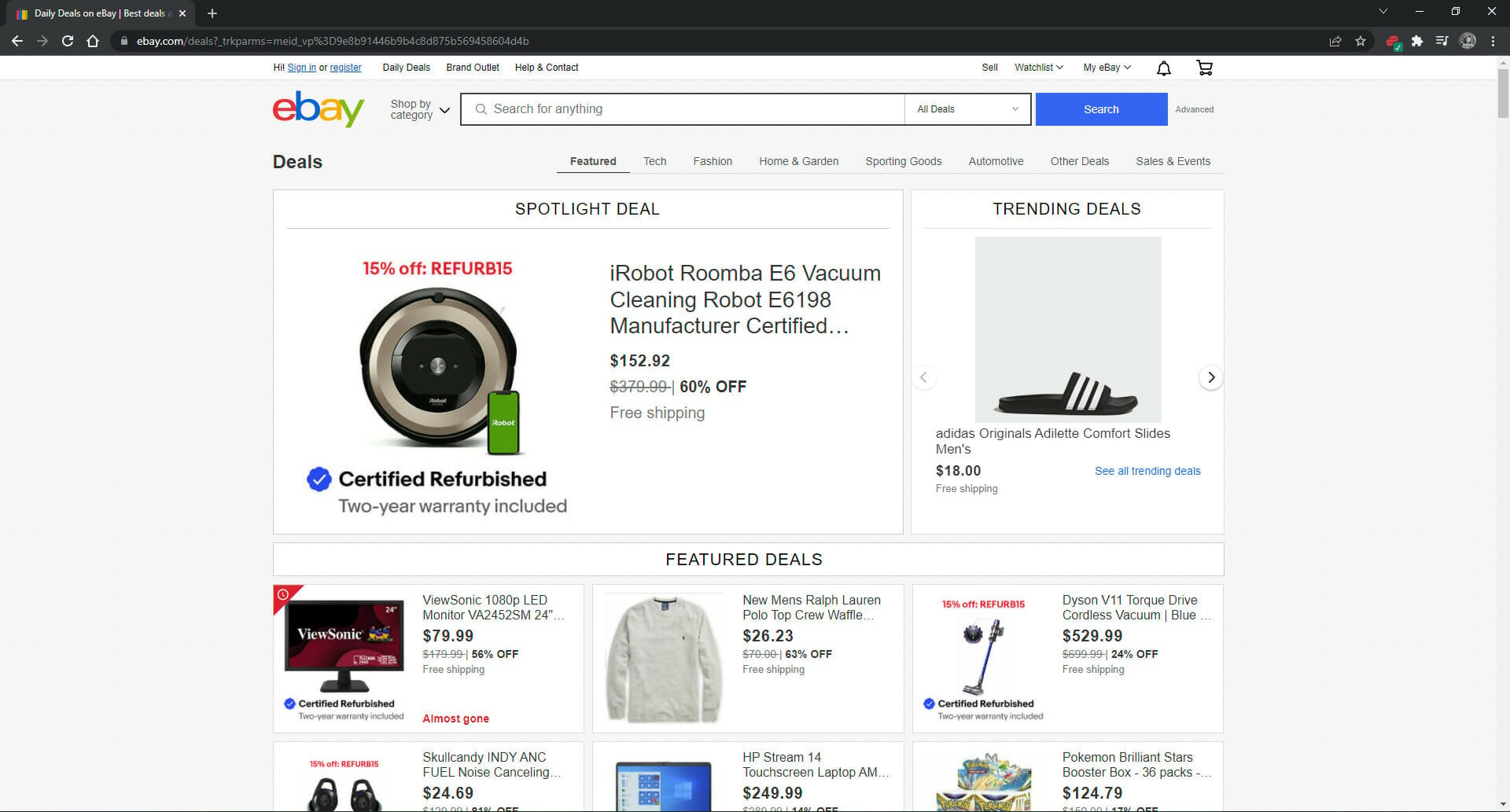In this snapshot of an open web page on eBay, we see the familiar red, blue, yellow, and green logo, and the text "Shop by Category" is prominently displayed. The search bar reads "Search for anything" with an empty field and a blue search button beside it. 

Highlighted in the "Spotlight Deal" section is a refurbished and certified Ruma vacuum cleaning robot available for $152.92, a significant markdown from its original price of $379. This deal includes free shipping, indicating a 60% discount.

In the "Trending Deals" section, several products are featured:
1. Adidas Originals Adilette Comfort Slides for men, priced at $18.
2. A Sonic TV or Monitor (apologies for the confusion in identifying it as a TV or monitor) available for $79.99.
3. A new Men’s Ralph Lauren polo top listed at $26.23, which appears to be a simple design rather than a quarter-zip style.
4. A Dyson Torque Drive cordless vacuum, distinguishable by its sleek blue design, priced at $529.99.

On the bottom row, we find a range of items:
1. Skullcandy Indy Fuel noise-canceling headphones.
2. An HP Stream 14 touchscreen laptop.
3. A Pokémon Brilliant Stars booster box on sale for $124, drawing particular attention due to its high value.

These visually engaging deals underline the diverse product offerings and significant discounts available, underscoring eBay's appeal to a broad range of shoppers.